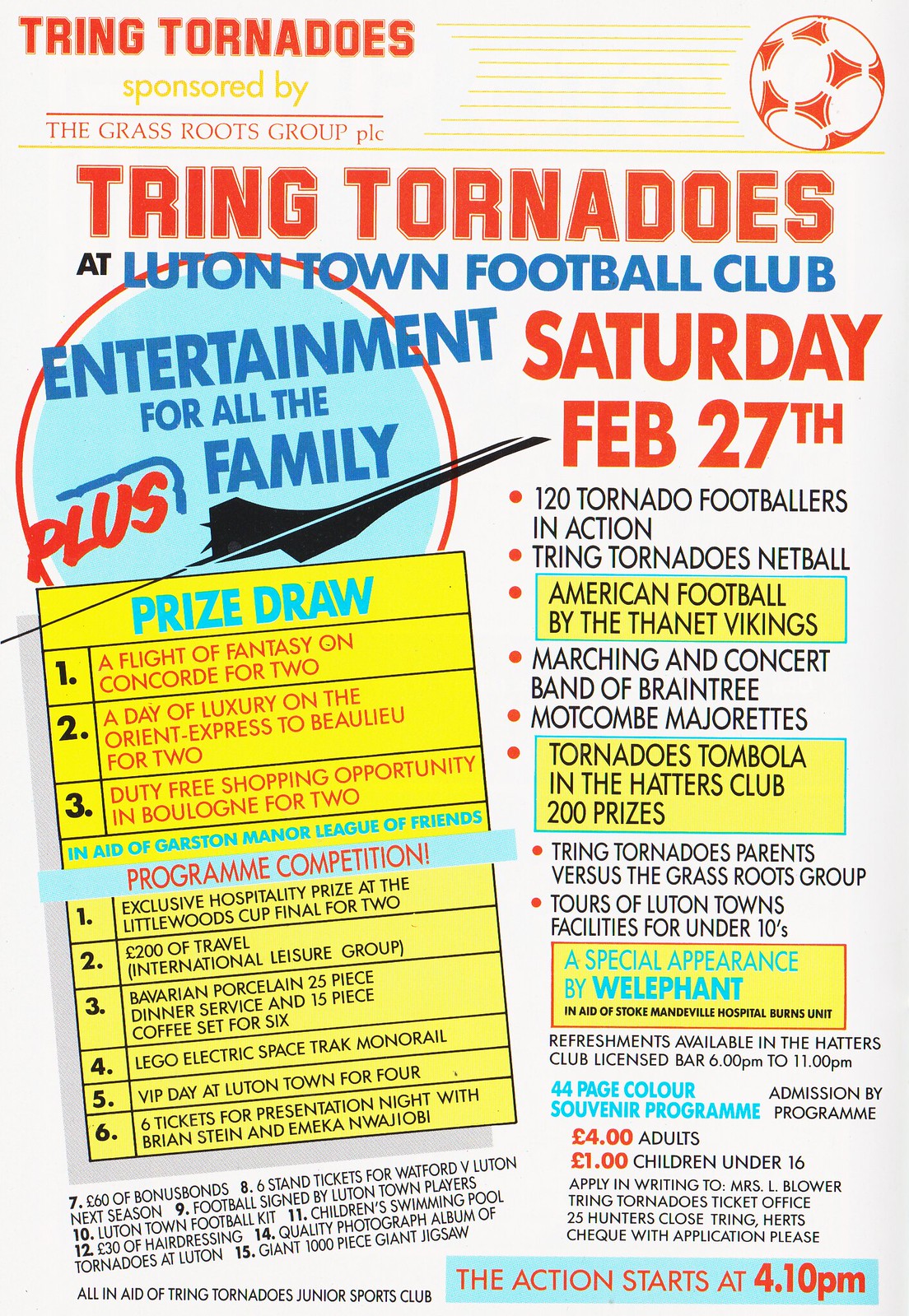This vibrant and densely packed poster announces a special event hosted by the Lutton Town Football Club, featuring the "Tring Tornadoes," sponsored by the grassroots group PLC. The header prominently showcases "Tring Tornadoes" in bold red print, with "at Lutton Town Football Club" in blue below it. A red soccer ball is located in the upper right corner, and a striking Concorde jet flies across a blue circle, symbolizing family entertainment.

The left column highlights a prize draw card offering luxurious prizes: a Flight of Fantasy on Concorde for two, a day on the Orient Express for two, and duty-free shopping. Additional prizes include exclusive hospitality for the Littlewood Cup finals, 200 pounds of travel, Bavarian porcelain sets, a Lego electric space track monorail, and a VIP day at Lutton.

On the right side, in bold red text, the date of the event is emphasized: Saturday, February 27th. A bulleted list details the activities:

- 22 footballers in action
- Tring Tornadoes netball
- American football by the Phalanx Vikings
- Marching Band and Majorettes
- Tornado Tumbles at the Hatters Club
- Tring Tornadoes parents vs. grassroots group
- Tours of Luton Town's facilities

Ticket prices are listed at the bottom: 4 pounds for adults and 1 pound for children, with the action starting at 2 PM. Set against a white background with colorful text in red, black, and blue, this busy poster is filled with details about an exciting family day out.